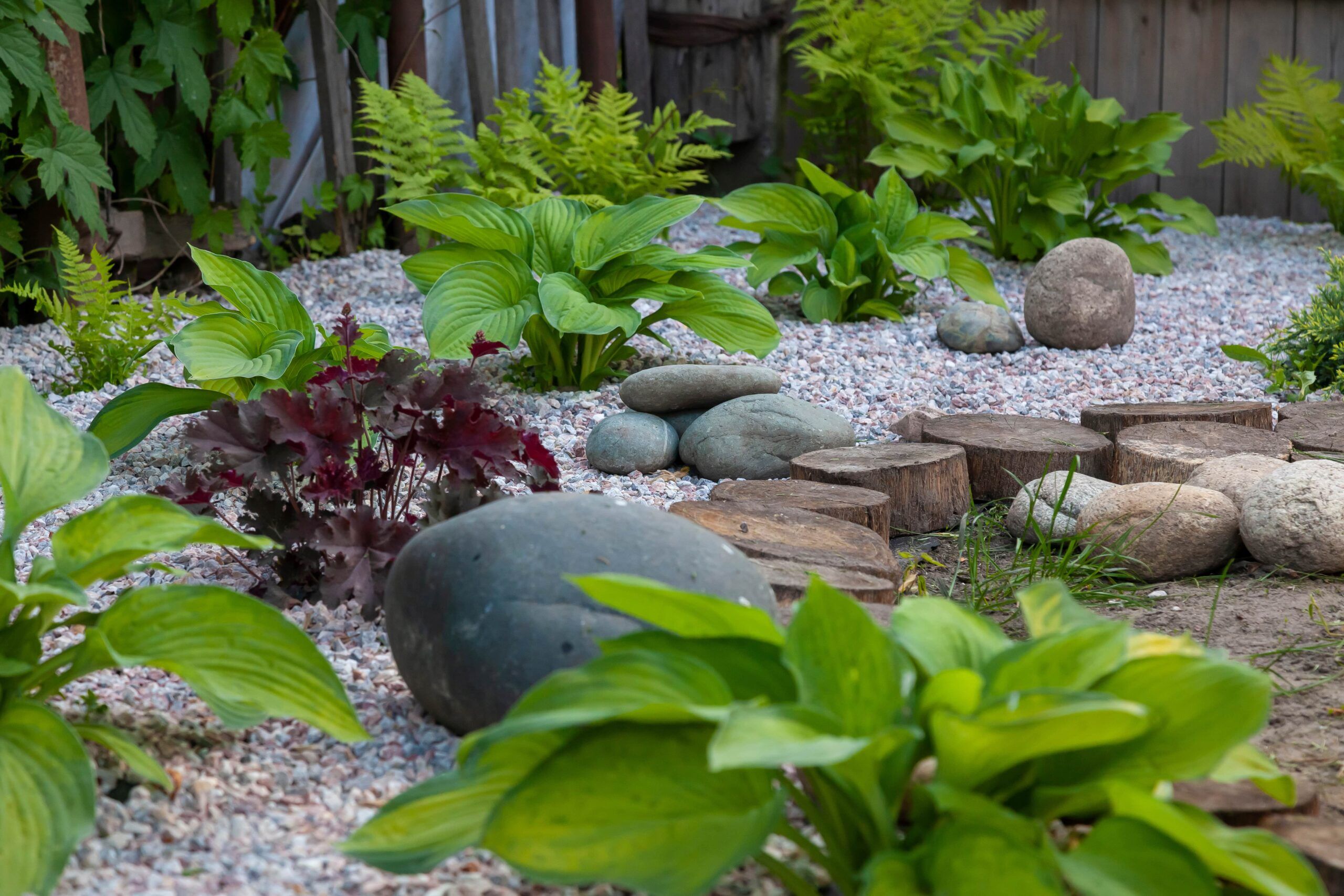This photograph captures a tranquil, zen garden that emanates a sense of calm and relaxation, seemingly designed as a personal escape. The garden, depicted from a low vantage point, reveals an intricately manicured space filled with various elements. The garden floor is composed of a mixture of white, orange, and light blue pebbles, with scattered rock formations of darker gray and tan tones.

Lush, green hibiscus-style plants with large leaves are strategically planted throughout the stone garden, numbering around 10 or 12. Additionally, a striking purple-leafed plant stands out among the greenery. Towards the back of the garden, ferns and ivy climb up a wooden fence, which frames the idyllic scene.

To the far right of the image, the garden transitions to a dirt ground dotted with large, circular stones. This area is bordered by approximately six or seven wooden stumps that separate the dirt path from the pebbled stone path. River rocks placed near the borders add to the decorative appeal. The entire garden is adorned with both green and red-leafed foliage, contributing to the vivid tapestry of colors. The meticulous arrangement of plants, stones, and wooden elements against the backdrop of the fence creates a serene and aesthetically pleasing environment.